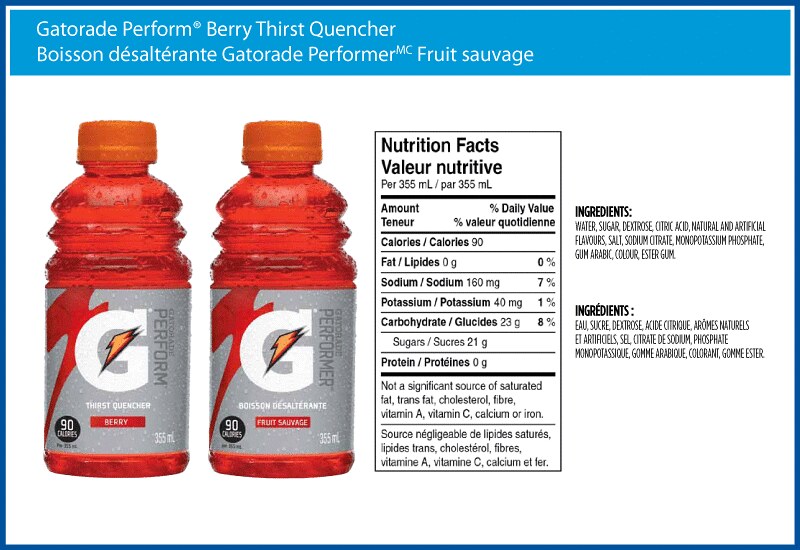The image is an advertisement for Gatorade featuring two red bottles filled with red liquid. Set against a blue rectangular background with a white interior, the ad prominently displays a large cyan-colored banner at the top that reads "Gatorade Perform" in white text, along with a copyright symbol. Below this, the text reads "Barry Thirst Quencher" and its French translation "Boisson désaltérante." 

Each bottle has a grey label featuring a large white "G" with an orange lightning bolt running through it. The left bottle is labeled "Barry" while the right bottle is labeled "Fruits Sauvage," both in white text on a red stripe. The blue border around the ad gives it a distinct frame. 

Additional details include a nutrition label and a section listing ingredients in both English and French. The label also highlights that each bottle contains 90 calories.